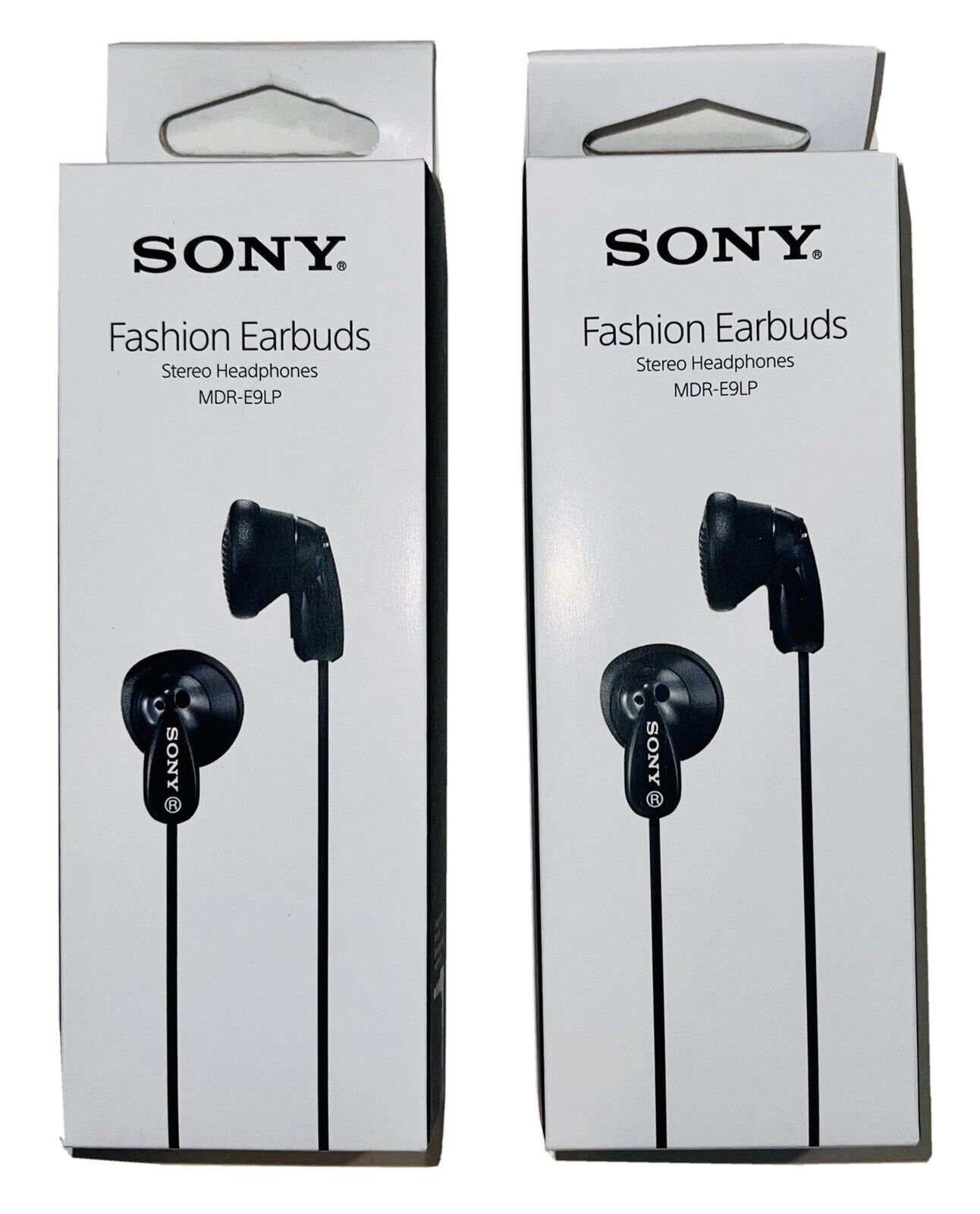This photograph, taken against a white background, features two identical boxes placed side by side, each showcasing Sony Fashion Earbuds Stereo Earphones MDR-E9LP. The boxes are taller than they are wide, with the Sony logo prominently displayed at the top in a larger font, followed by the product description in smaller black text. Each box, otherwise white, includes an image of the same pair of black wired earbuds. The earbud on the left side of the image displays the Sony logo and an "R" indicating it is for the right ear, while the earbud on the right is presented from a side angle. A thin wire extends from each earbud down to the bottom of the box. The identical layout and graphics make the two boxes appear as mirror images in the photograph.